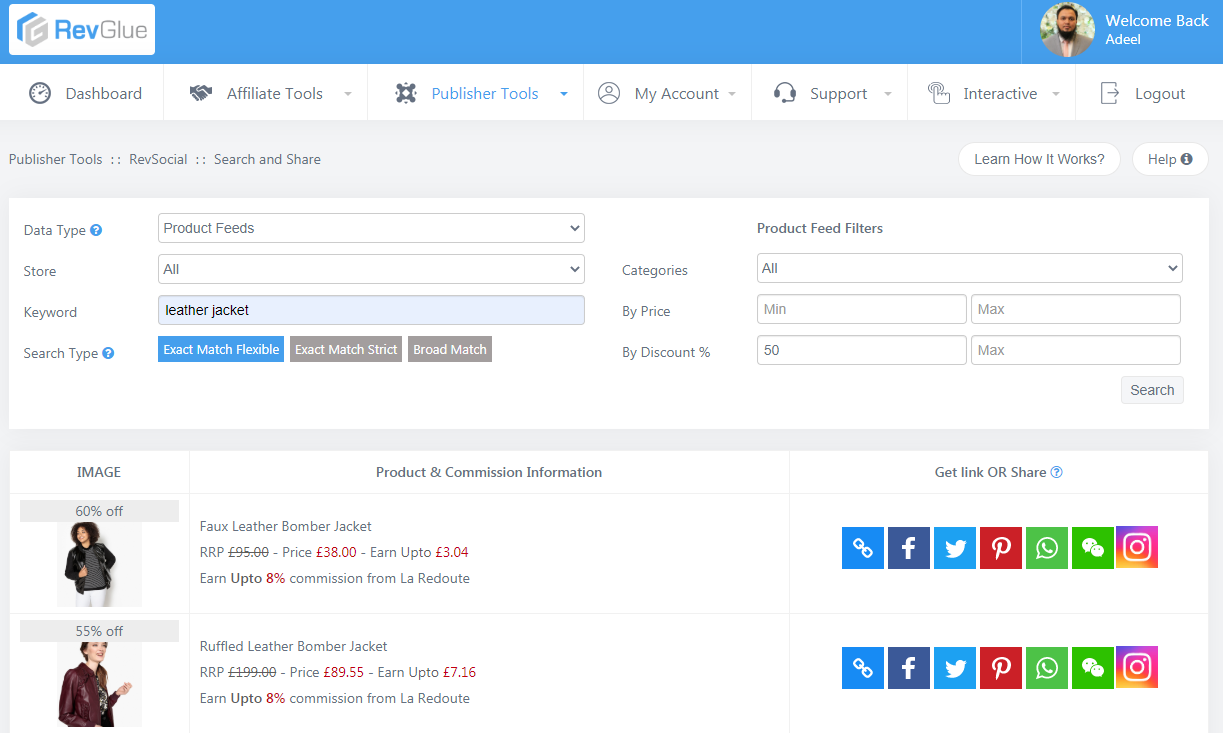**Descriptive Caption:**

The website page is organized with a sky-blue header running horizontally across the top. In the top left corner of the header, there's a white box with a gray "G" partially outlined in blue, representing the logo. To the right of the logo, the company name "Rev Glue" is displayed, with "REV" in blue and "GLUE" in gray.

On the far right of the header, a circular profile picture depicts a man with light brown skin, black hair, and a black beard. He is dressed in a gray jacket and pink tie. Next to his photo, the white text reads "Welcome Back" followed by "ADEEL."

Below the header, a navigation bar features several icons and labels:
1. A clock icon labeled "Dashboard" in black.
2. An indistinguishable black avatar icon with the label "Affiliate Tools."
3. A gear icon labeled "Publisher Tools" in blue.
4. A circle icon with a person figure labeled "My Account" in black.
5. A headset icon labeled "Support" in black.
6. Another indistinguishable black avatar icon labeled "Interactive."
7. A book icon labeled "Logout" in black.

Further down, on the left, the section labeled "Publisher Tools" includes several sub-options:
1. "Ref Social" with a four-dot box icon.
2. "Search and Share" with another four-dot box icon.

To the right of these options, there are two search bars with placeholder texts:
1. "Learn How It Works" in the left-hand bar.
2. "Help" in the adjacent bar.

Under these, a form is provided to input various data points:
- Data Type
  - Product Feeds
- Store (with a search bar labeled "All")
- Keyword (with a search bar containing "Leather Jacket" in black)
- Search Type
  - Three options: "Exact Match Flexible" (blue with white text), "Exact Match Strict" (gray with white text), and "Broad Match" (gray with white text)

To the right, under "Product Feed Filters," search options include:
- Categories (with a search bar labeled "All")
- By Price (with two search bars: "Minimal" and "Max")
- By Discount % (with two search bars: the first defaulted to "50" and the second to "Max")

The "Search" button is located below these filters.

At the bottom of the section, the "Product and Commission Information" area displays two images stacked vertically:
1. A woman with curly dark hair wearing a black leather jacket over a gray and black shirt.
2. A Caucasian woman with brown hair pulled up, wearing a maroon leather jacket over a black and white shirt.